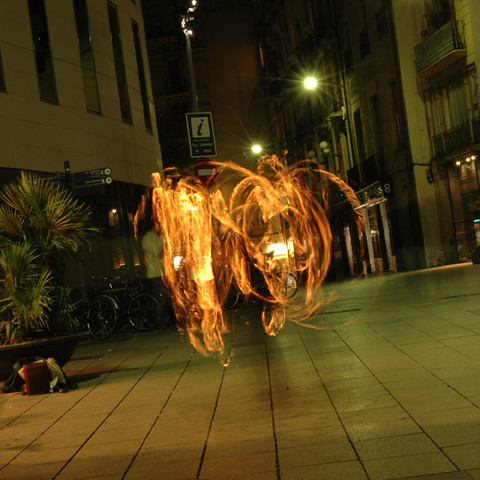This perfectly square photograph, set at night, captures a mesmerizing scene of a person spinning fire in the center of a paved pedestrian street made of square stone tiles. The long exposure of the spinning fire creates enchanting yellow and orange circular patterns, giving the impression of an art installation rather than a fluid motion. The person, dressed in a long-sleeve shirt and black pants, wields black rods with lights or flames at their ends, contributing to the fiery spectacle. The backdrop reveals a dimly lit urban environment, with several streetlights illuminating white and brown multi-story buildings adorned with windows and signs. On the left side of the image, plants and bushes frame the scene, along with some potted plants and bicycles. The sky is black, delicately accented by thin, wispy white clouds, grounding the photograph in a serene yet dynamic nocturnal setting.